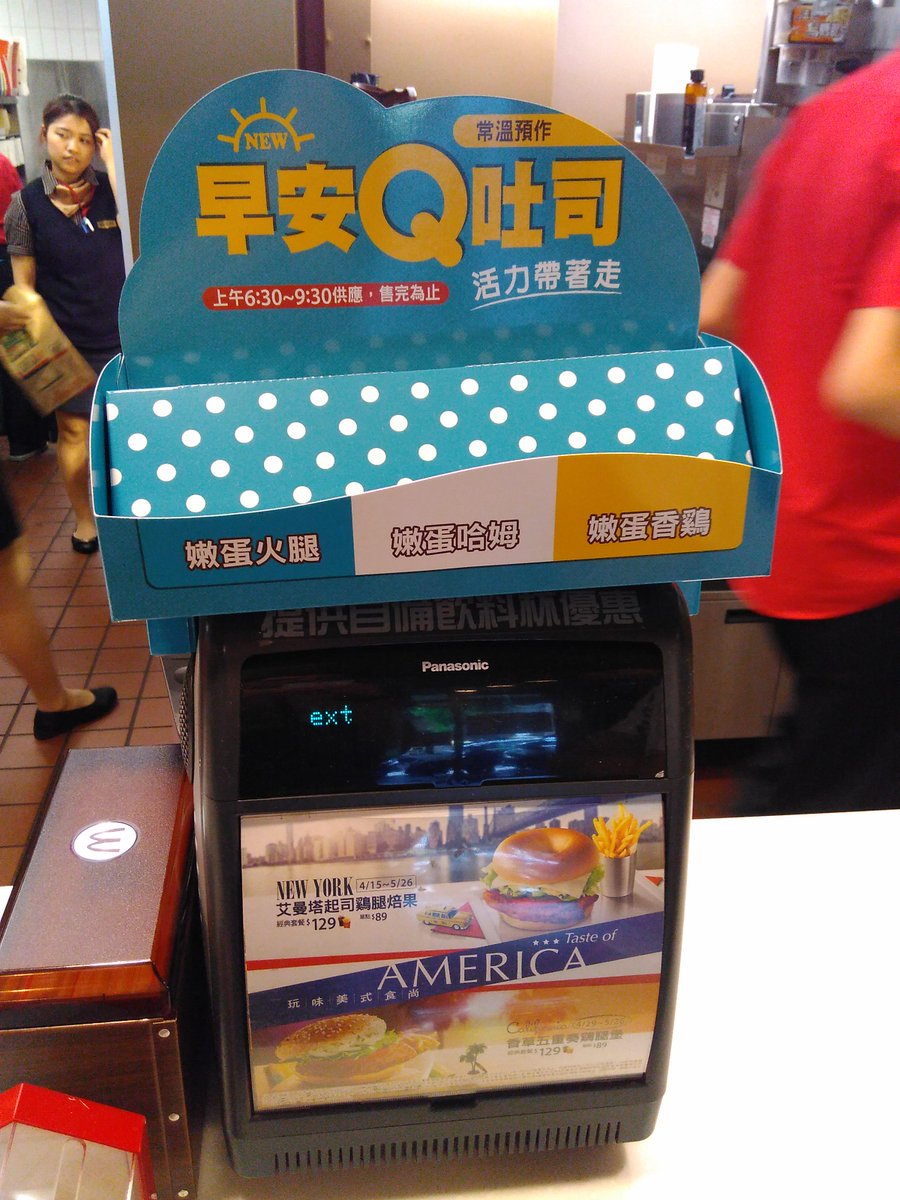In this vibrant image of a bustling food shop, various elements come together to create a lively scene. At the bottom center, a sleek Panasonic machine prominently displays a colorful and enticing advertisement, showcasing a burger with the tagline "Taste of America" alongside imagery of pizza and fries. Towards the top left of the image, a woman, seemingly deep in thought, scratches her head. On the right side, a man dressed in a red shirt and black trousers appears to be engaged in the activity around him. The color palette of the scene is dominated by hues of blue, white, red, black, and yellow, adding to the dynamic atmosphere of the shop.